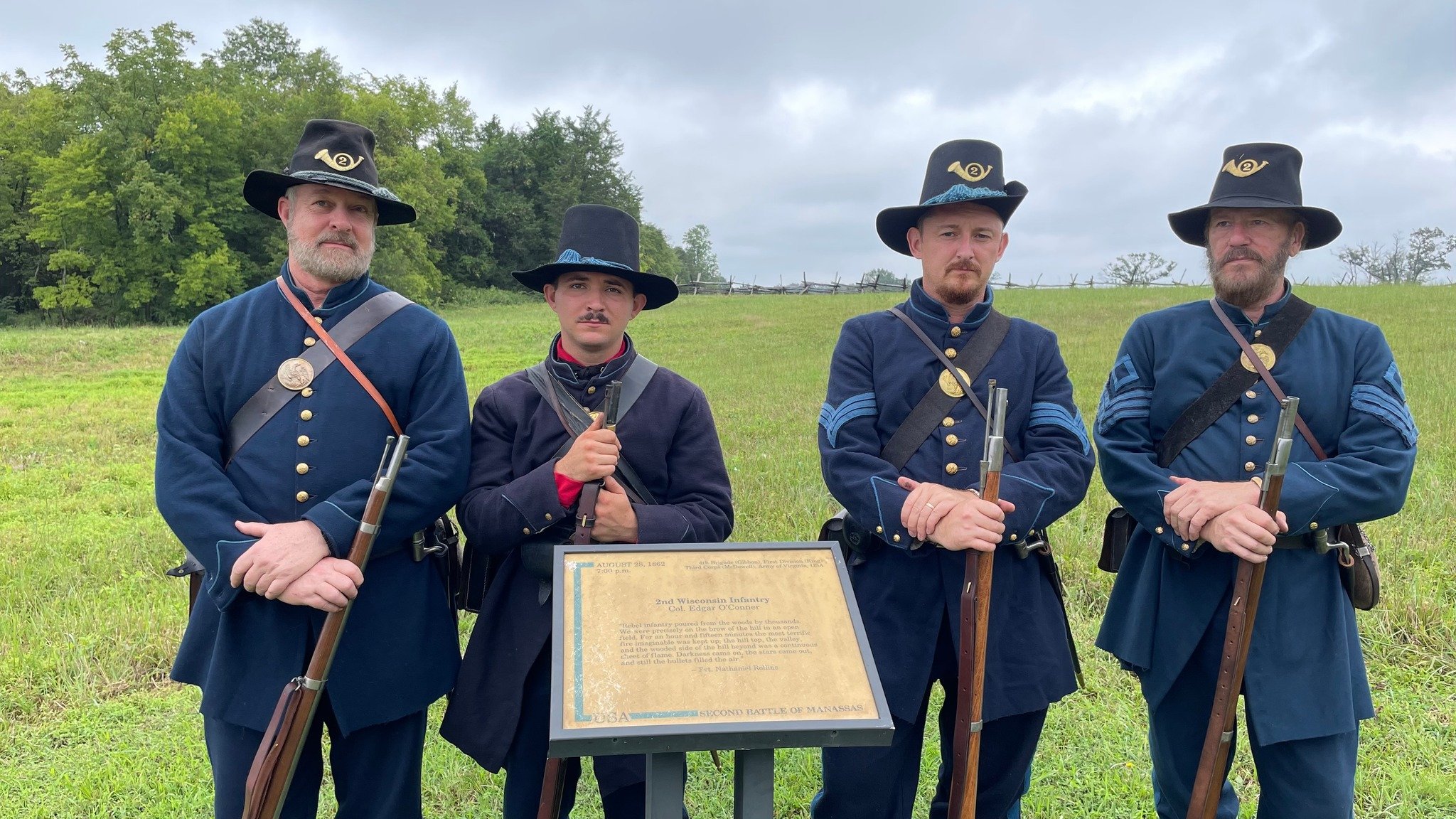In this photograph, four white men, dressed as Civil War reenactors, are standing in a green field under a cloudy sky, with trees in the background. They are positioned in front of a gold-colored plaque on a wooden stand, the text on which is indiscernible. Each man holds a 19th-century style musket, adding historical authenticity to their portrayal. Three of them wear matching blue military uniforms adorned with gold buttons, light blue stripes, and soldier's hats with wide bills featuring trumpet symbols. The first man, a tall individual with a beard, stands with his hands crossed. The second man, shorter and only sporting a mustache, looks directly at the camera. The third man, equally tall but thinner than the first, also has crossed hands. The fourth man, the oldest with a graying beard, diverges by wearing regular clothing and not looking at the camera. Their detailed uniforms, complete with a gold circular plate on a sash across their chests, enhance the historical reenactment scene they are likely about to perform or have just concluded.